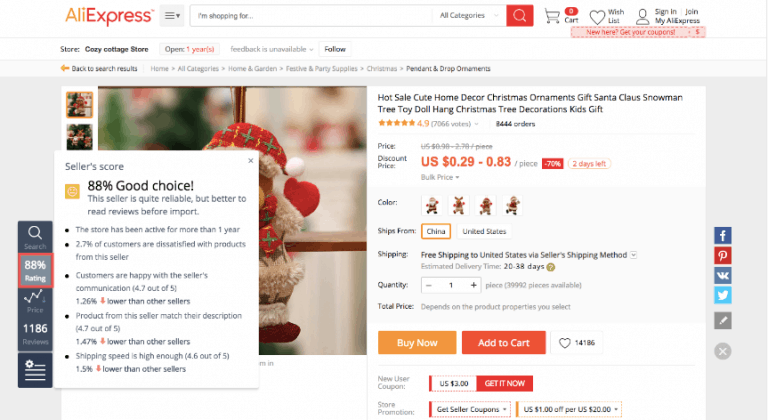This cropped screenshot showcases the desktop version of the Aliexpress website featuring a product listing. At the top left, the Aliexpress logo is prominently displayed against a white header. Adjacent to the logo is a search box with placeholder text "I'm shopping for," followed by a dropdown menu labeled "All Categories" and a red search button with a magnifying glass icon. To the right of the search box, there is a cart icon with a red notification bubble indicating "0" items, followed by a wishlist icon, and a profile icon next to the text "Sign in or Join."

Immediately below the header, the section titled "My Aliexpress" is visible. Underneath, the store information is displayed, showing the store name and status "Open," with "1 years" in red font indicating the store has been active on Aliexpress for one year.

Beneath this, the main product listing begins, although the left side is partially obscured by a large white pop-up box stating "Seller Score, 88% good choice." To the right of this pop-up is a vertical gray rectangular banner. This banner features a search option at the top, highlights the 88% rating within a red box, and includes additional options below.

To the far right, the full product listing is visible. The product titled "Hot Sale, Cute Home Decor, Christmas Ornaments, Gift, Santa Claus, Snowman, Tree, Toy, Doll, Hang, Christmas Tree Decoration, Kid's Gift" is detailed. It displays a seller rating of 4.9 stars and the product price. The listing includes thumbnails showcasing different colors, a "Ships From" option with China selected (alternatively, the United States can be chosen), and details about shipping. Below this, there is a quantity selection box and a total price section that currently does not list a price. At the bottom left, two buttons are available: an orange "Buy Now" button and a gray "Add to Cart" button.